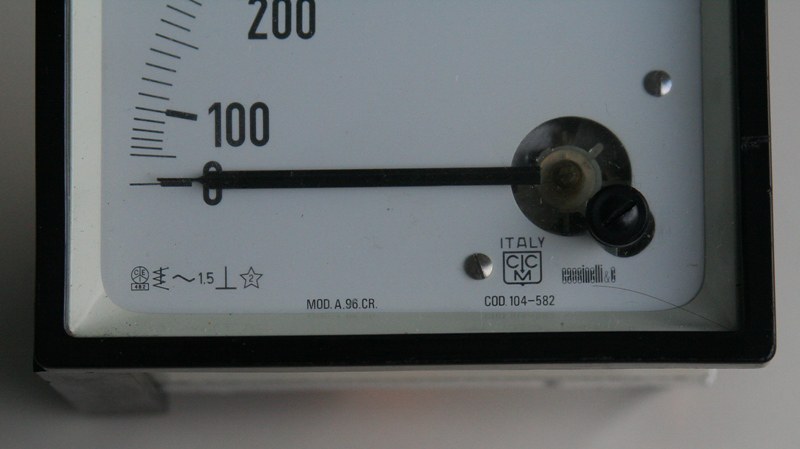The image showcases the bottom portion of a food scale with a stainless steel and black trim. The scale features a white circular face with numerical increments in hundreds, prominently displaying the numbers 100 and 200. To the right side of the scale, there is a black adjustment knob. Beneath the knob, the word "Italy" is inscribed, followed by a boxed notation "C-C" with an "M" directly underneath it. Additionally, the code "COD 104-582" is visible on the right side of the scale. On the left side, there are various symbols accompanied by the label "M-O-D-A-9-6-C-R." The scale is either resting on a white surface or possibly mounted on a wall, though the precise setting is unclear from the image.